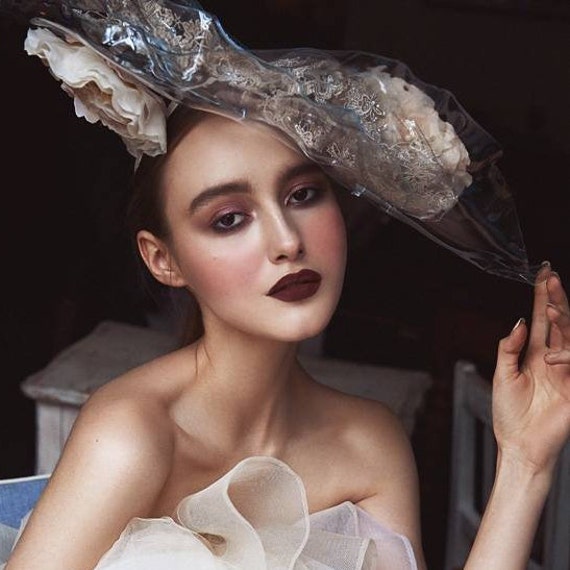In this evocative, square portrait image, a young woman in her early twenties gazes directly at the viewer. She sports a dark red, burgundy lipstick that complements her flawless makeup, including dark purple metallic eyeshadow and a smoky eye effect, accentuated with delicate blush on her cheeks. Her light brown hair is elegantly tied back in a ponytail. She wears an off-the-shoulder, strapless white dress made of fluffy chiffon material. A distinctive, large hat adorns her head, tilted at a 45-degree angle. The hat is crafted from a unique, transparent material with a wrinkled texture reminiscent of a Kentucky Derby style, featuring two prominent white flowers affixed to both the top and underneath the brim. Her left hand is gently touching the brim, emphasizing the intricate detail of the hat. The backdrop is a nearly black, dark room with minimal discernible furniture, including a light grey wood desk and chair, which subtly frame the elegant figure of the woman.